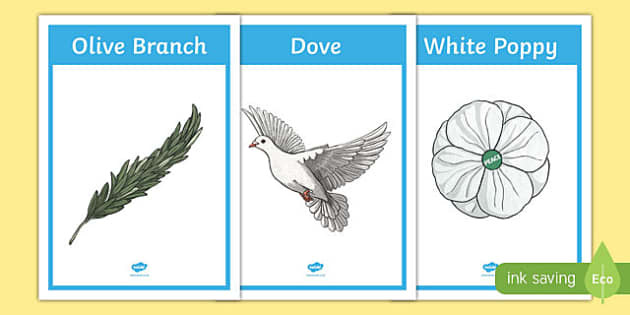The image features three vertically aligned rectangular cards overlapping slightly from left to right, each with a distinct design and detailed illustration. All cards share a white border with an inner blue-lined box and a blue banner at the top displaying white text. The first card, on the far left, is labeled "olive branch" and depicts a dark green olive branch angled from the bottom left to the top right. The middle card, labeled "dove," shows a white dove mid-flight, facing left, with orange beak and feet and wings spread wide. The rightmost card is labeled "white poppy," illustrating a poppy flower with white petals and a green center. Below each illustration, in a small green banner located at the bottom right, is white text that reads "ink saving eco." Each card also features a small, subtle blue and white logo at the bottom. The background of each card appears to be a soft yellow, enhancing the visibility of the white borders.